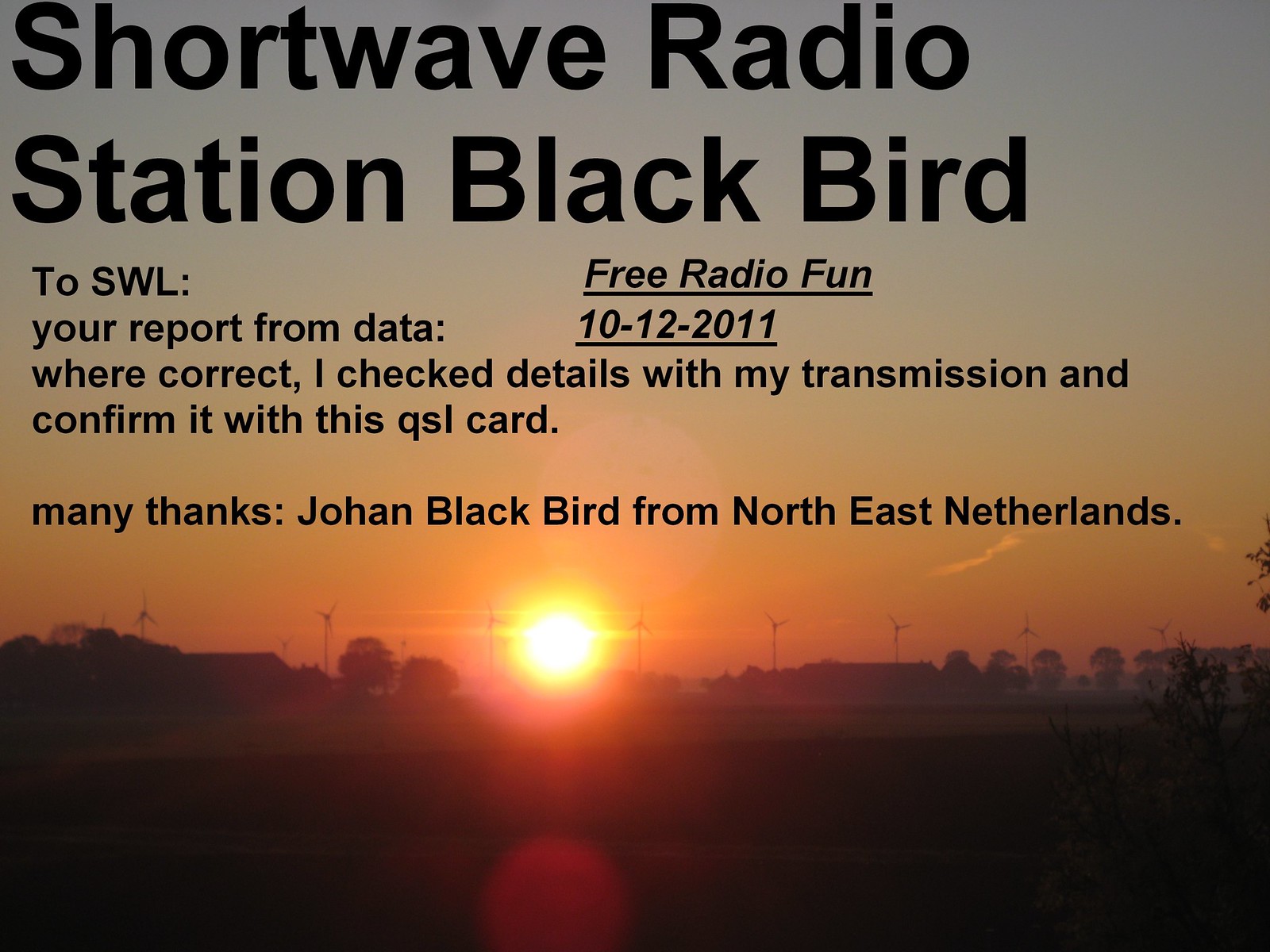The image captures an outdoor scene during sunset, where the Sun is a bright yellow orb descending close to the horizon. The sky features a gradient from orange to gray with a few small clouds scattered throughout. Silhouetted against the dusk sky are several three-pronged windmills. The lower part of the photo is shadowed, making the landscape, which includes some buildings and trees, nearly dark. Prominent black text at the top reads "Shortwave Radio Station Blackbird" in large letters, with "Free Radio Fun, 10-12-2011" underlined beneath it. Smaller text below includes the message: "Your report from the data was correct. I checked the details with my transmission and confirmed it with this QSL card. Many thanks, Johan Blackbird from Northeast Netherlands."